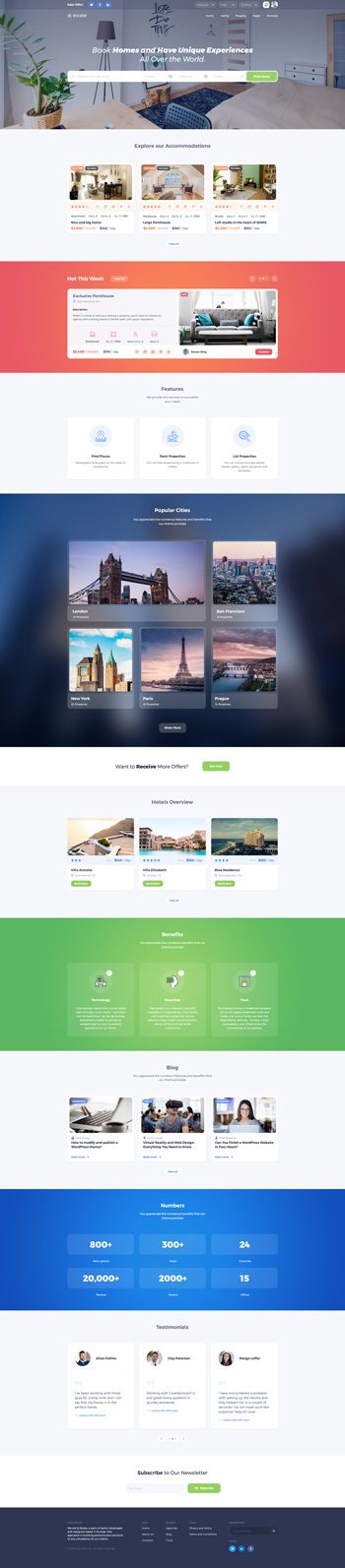At the top of the image, there is a section depicting the concept of book homes and the unique experiences they offer around the world. This section features a bold green rectangle and includes three pictures of different types of stars. Below this, a red rectangle is labeled "How This Works", accompanied by several photos and three images highlighting popular cities. The background is a vibrant purple, showcasing iconic landmarks such as the London Bridge, various buildings, and the Eiffel Tower.

Further down, there is another green rectangle containing three pictures, followed by an additional green rectangle with three squares that feature different icons and accompanying text. As we continue, we see more images and statistical data: 800+, 300+, 24, 20,000+, 2,000+, and 15.

The testimonials section has a prominent layout with black text. On the left side, there is a square with a person's image at the top left and text in the middle. The right side also includes text and another person's image at the top.

Towards the bottom, there is a call to action to "Subscribe to our Newsletter," displayed inside a green oval. At the very bottom, a dark bar contains links to social media platforms including Twitter, Facebook, and LinkedIn.